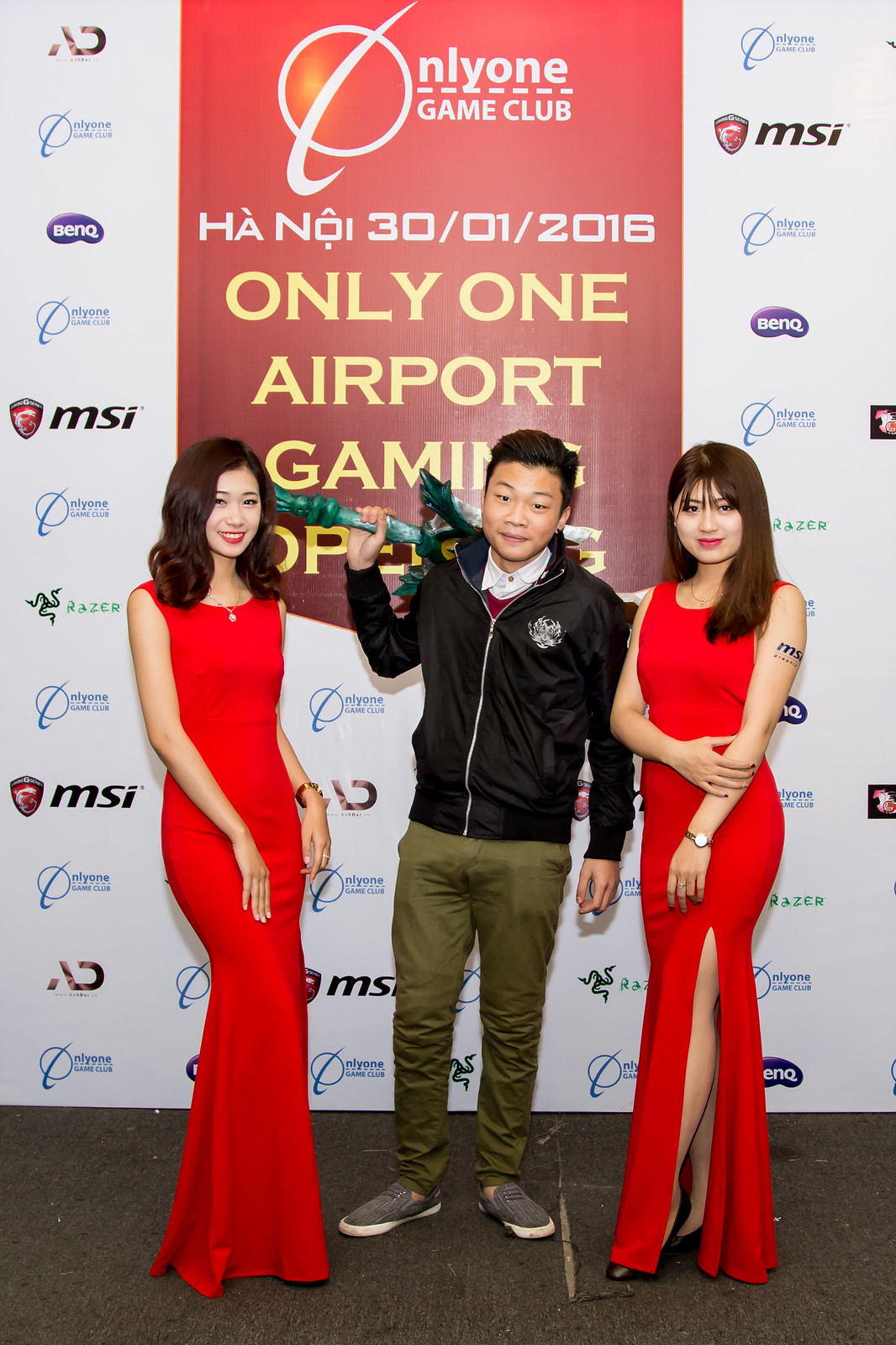The image captures three people of Asian descent standing in front of a step-and-repeat backdrop at an event titled "Nylon Game Club, Hanoi 30-01-2016, Only One Airport Gaming Opening." The backdrop features various logos from sponsors such as MSI, BenQ, and OnlyOne, along with other logos in Asian characters. Central to the photograph is a casually dressed man with green pants, a black track jacket sporting a logo, a white shirt, and a red sweater underneath. He is notably holding an object behind his back that resembles a dragon's tail or a toy sword with green wings. Flanking him are two women in formal, sleeveless red gowns; the woman on the right appears to have a tattoo or an advertisement on her upper arm. The man and the women strike a pose against the white, logo-filled background, standing on a floor with a dark-colored rug.